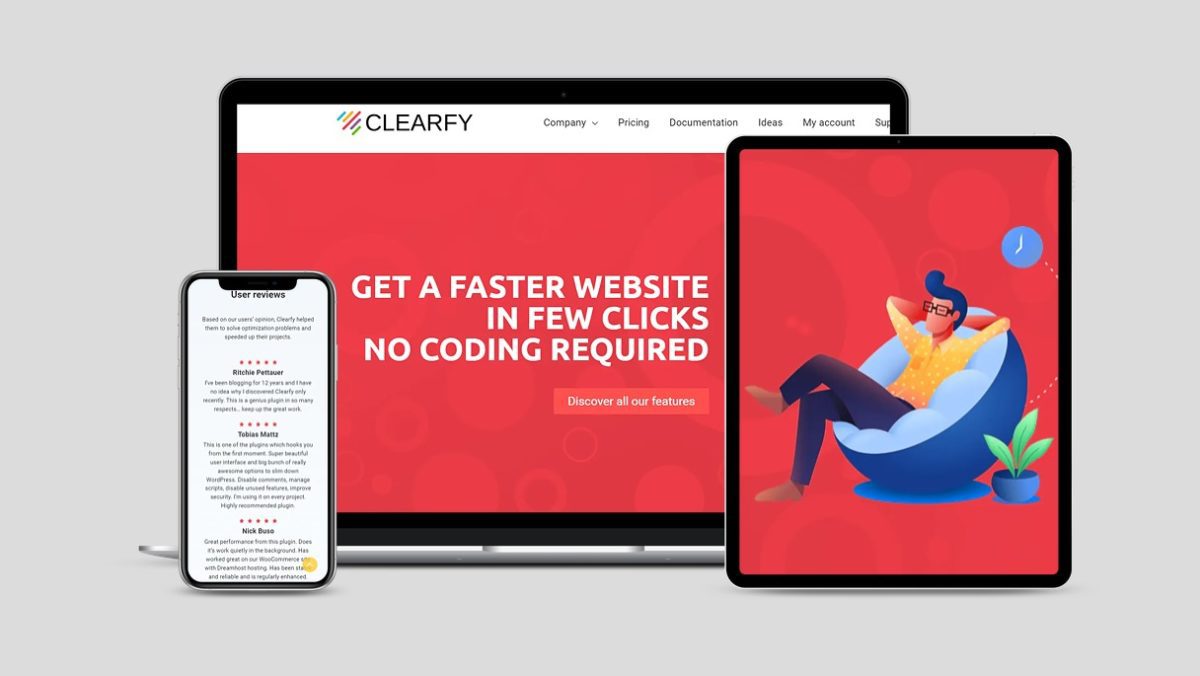The image depicts a neatly arranged workspace featuring a cell phone, a computer, and an iPad, all positioned beside each other. On the far left is the cell phone displaying a screen with "User Reviews" and three individual reviews listed below. At the center is the computer screen, prominently showing a webpage titled "Clarify," with dropdown menus related to company pricing, documentation, ideas, and account details. The screen also highlights a promotional message stating, "Get a faster website in a few clicks, no coding required," followed by "Discover all of our features." On the far right, an individual sits in a modern, egg-shaped chair with their legs crossed and hands placed behind their head, creating a relaxed pose. The person is wearing glasses and appears to be unwinding. Beside the chair, there is a plant with three green leaves, housed in a stylish blue and navy plant stand, adding a touch of nature to the setup.